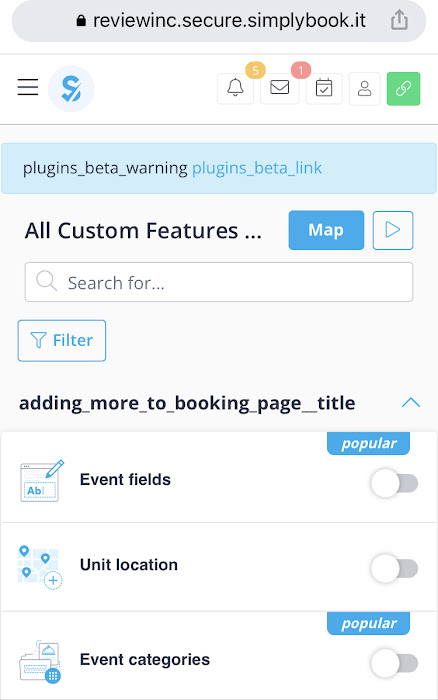This image is a screenshot from a mobile device displaying a user interface, likely from a booking or scheduling application. At the top, there's a grey bar with the URL "review.inc.secure.simplybookit." On the left side of this bar, there are three horizontal lines, which appear to be a menu icon. Adjacent to this icon is a symbol resembling a dollar sign, although it might represent something else due to its unique design with hash marks.

On the right side of the grey bar, there are several icons: an alert icon with the number "5" next to it, indicating notifications; an envelope icon marked with "1," likely for emails; a calendar icon; a person icon; and a green lock icon, which could signify a security feature or user authentication.

Below the grey bar, there is a blue box with the text "Plugins, Beta Warning." Following this, on a white background with black text, there is the heading "All Custom Features." To the right of this heading, there's a button labeled "Map," indicating it can be pressed to access a map feature. Below this, there is a search box and a filter box.

Further down, there are sections labeled "Event Fields," "Unit Location," and "Event Categories." Each of these sections has corresponding buttons on the right, which can be toggled on or off. Currently, all the buttons appear to be in the off position. Above the "Event Fields" and "Event Categories" buttons, there is a label "Popular" in blue and white text, indicating these features might be frequently used.

The overall background is predominantly white, giving the interface a clean and minimalist look.